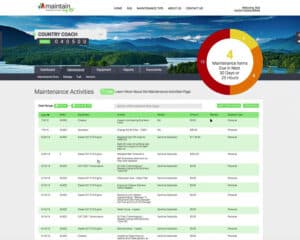This image depicts a smaller, zoomed-out view of a website situated against a white background, although no visible borders can be discerned. In the top left corner of the website, there is a page title accompanied by a small symbol. Centrally aligned are five selectable options or names. Over on the right-hand side, two lines of text are visible, one above the other. 

Below these elements, a prominent rectangular image showcases a scenic view of mountains and trees. Superimposed on this scenery is a large circle featuring the number '4' with its edges colored in a gradient of red, orange, and yellow. Beneath the scenic image, a title appears, likely related to activities.

Further down the page, there is a partially visible document, segmented into several rows. These rows alternate in color between dark green, light green, and white at the top, transitioning to a repeating pattern of light green and white lower down.